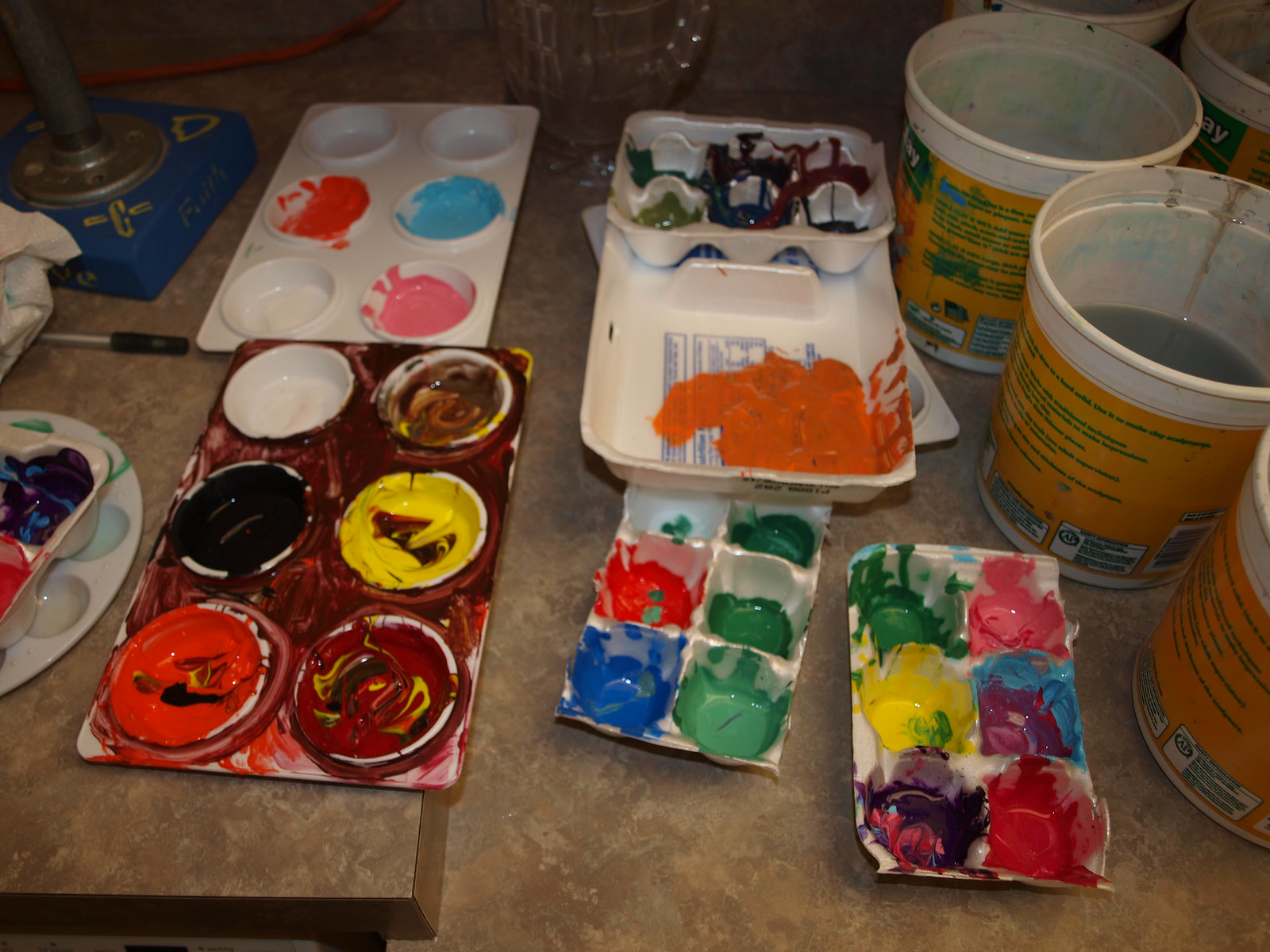The image displays an assortment of paint trays, each spattered and filled with various hues of paint, indicative of recent or ongoing art projects. Prominently featured are four plastic trays with multiple indentations, designed to hold paint for easy access by artists. In addition to these, there is a makeshift paint tray fashioned from a cut-up egg carton, suggesting resourcefulness and improvisation.

Each tray shows a palette of mixed colors, including vibrant pinks, blues, oranges, purples, yellows, and greens, interspersed with more subdued browns and blacks. The chaotic blending within the trays reveals a creative explosion, with some colors distinctly pooling in certain sections while others bleed into each other.

Also present in the scene are several small plastic cups, yellow and white with green writing that is indecipherable. The cup interiors appear to contain murky water, likely used for rinsing paintbrushes.

Amidst the organized chaos of paint and tools, the surface underlain is a marble-brown countertop or possibly a similarly hued floor, serving as the backdrop for this vibrant display of artistic endeavor.